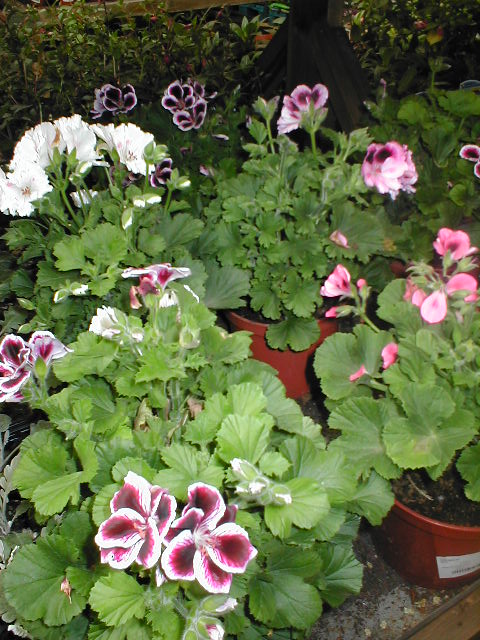The photograph showcases a vibrant, lush arrangement of potted flowers from a bird's-eye view. The plants are housed in orange-ish brown pots set on a gray concrete surface, although only parts of the pots are visible. Dominating the scene are the lush green leaves framing a spectrum of blooming flowers. Central to the image, the flowers display a striking gradient—white petals transitioning to neon pink, deepening into red, and finally to a dark center, with these flowers clustered together to form full, eye-catching blooms. Among these, some flowers possess vibrant pink hues, while others blend into deep pinks with purplish tones, adorned with white borders. In the foreground, noticeable are pots with adhered white stickers, particularly on the lower right side. The upper background reveals two long rows separated by a dark walkway, where additional clusters of green foliage and varied blossoms are slightly obscured by dim lighting. Overall, the image captures a rich tapestry of color and texture, highlighting the layered beauty and diversity of the potted garden.